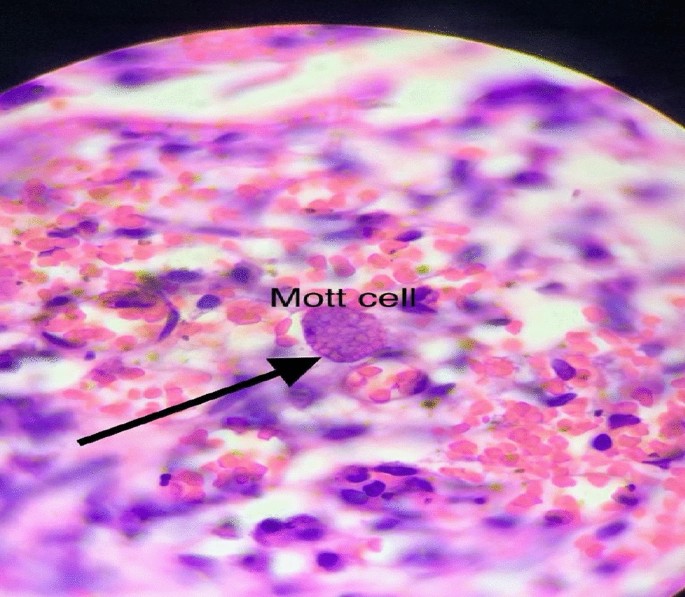This image appears to be a microscopic view of a biological sample, predominantly circular in shape with varying shades of pink, purple, and white. At the top of the circle, there is a subtle black curvature. The center of the image features the text "MOTT CELL" in black, accompanied by a black arrow pointing towards the middle. Surrounding this central area, numerous scattered pink bits and darker purple spots can be observed, giving the impression of a cellular or organic structure.